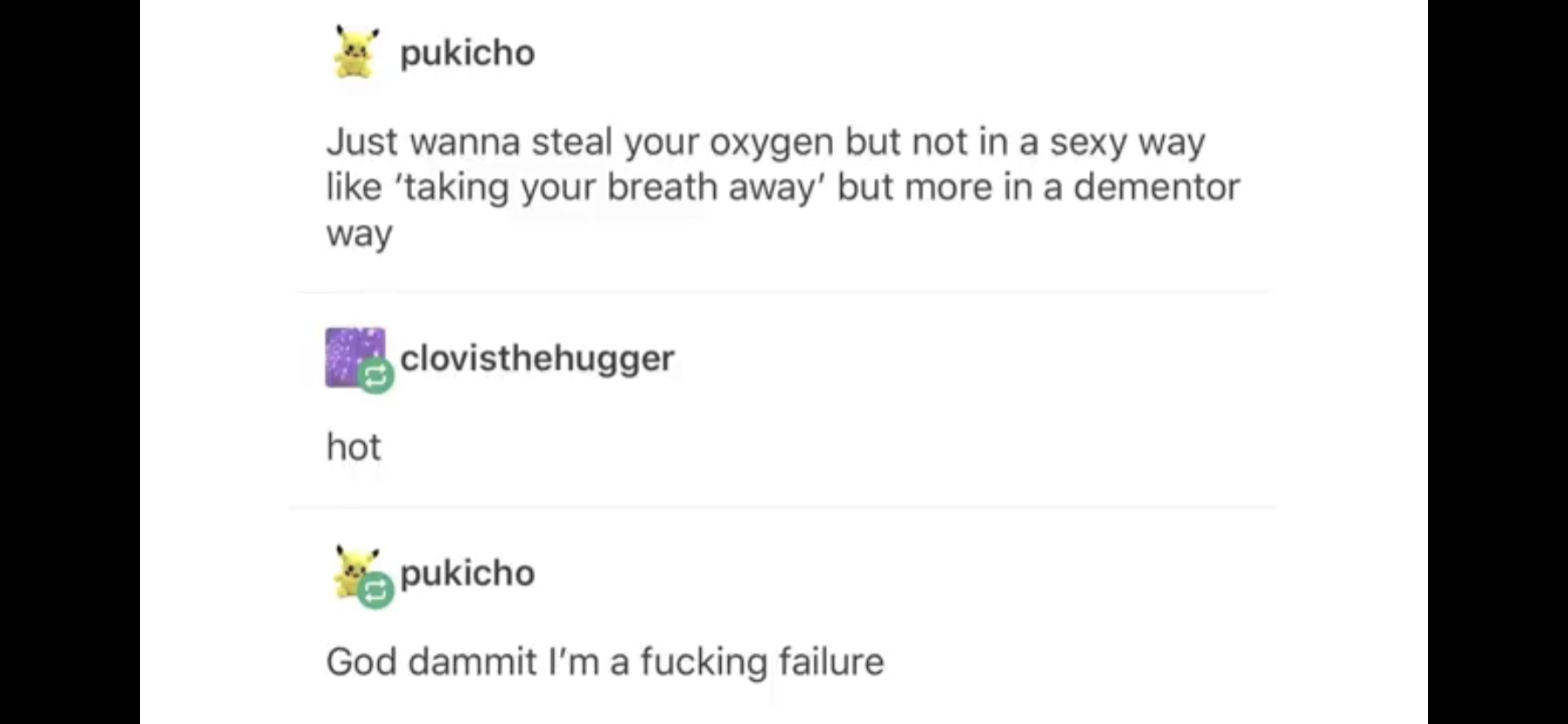The image is a color screenshot from a cell phone app or video game, displayed in landscape orientation. It features vertical black bars on both the left and right sides. At the center is a white text box with black text displaying a conversation between characters. The first icon is a yellow creature labeled "Pukicho" in bold black letters. Following this is a line of dialogue in black text that reads: "Just want to steal your oxygen, but not in a sexy way like taking your breath away, but more in a demented way."

Below this text is a response from another character, whose icon is a purple square with a green circle, labeled "Clovis the Hugger" with the accompanying description "hot." Underneath this is another post from the original poster with the yellow creature icon and green conversation circle labeled "Pukicho," followed by the text: "God damn it, I'm a fucking failure."

The image incorporates detailed and whimsical illustrations, emphasizing the quirky and irreverent tone of the conversation.